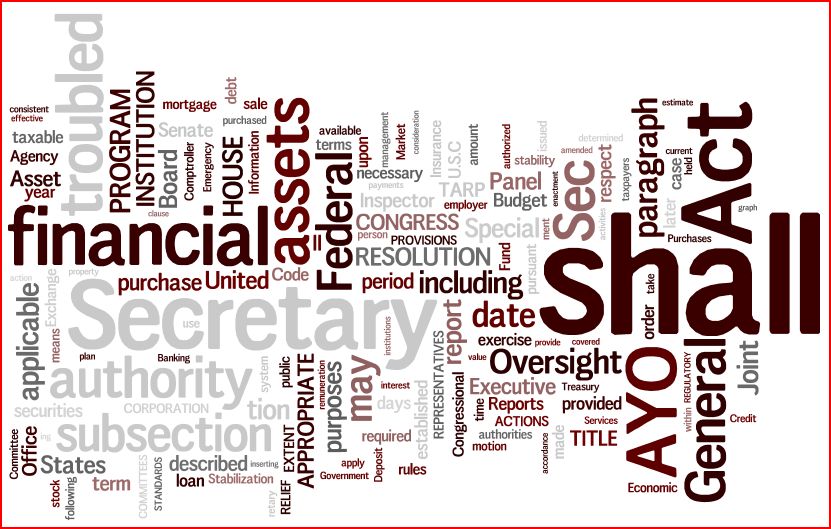The image appears to be an advertisement for a financial institution, presented in a visually striking and artistic manner. The paper is oriented horizontally, showcasing a collage of words jumbled together in various shapes, sizes, and directions. Some of the prominent words, highlighted in both black and gray, include financial, assets, federal, general, authority, applicable, and resolution. Additionally, terms like secretary, office, states, motion, executive, oversight, Congress, and board are also visible, suggesting connections to legal and political aspects. The overall design is neat and tidy, making it easy to see the words despite their scattered arrangement, but it lacks a clear direction or message.